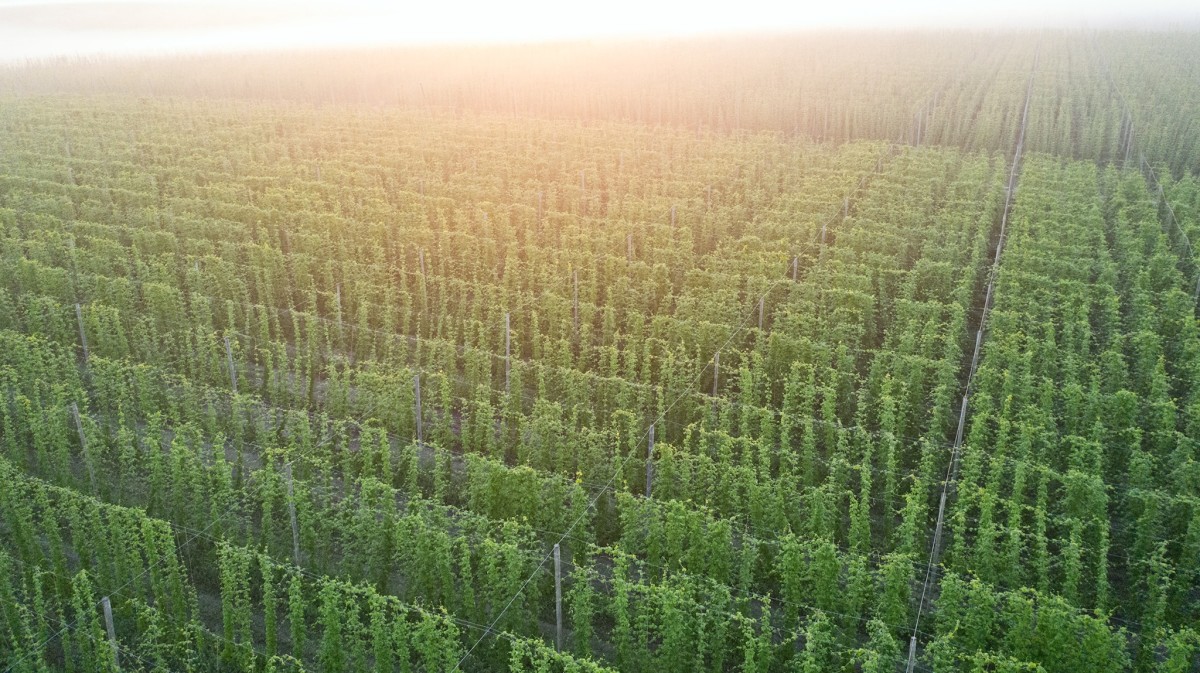This color photograph, taken from above in landscape orientation, offers an expansive view of a vast agricultural field, most likely a hop farm. The scene is bathed in the intense, captivating light of either sunrise or sunset, casting a pinkish-orange hue over the horizon and suffusing the plants with an orangish-yellow tint, especially towards the left side. The meticulously arranged rows of climbing plants are set on trellises that run diagonally across the image from the higher top left corner to the lower bottom right. These green, uniform vining plants extend for miles, creating a rhythmic pattern across acres of land.

The rows are interspersed with fence-like structures, consisting of vertical posts connected by netting or rope, which segment the farm into distinct sections. These barriers enhance the orderly appearance and possibly support the growth and structure of the plants, which require frames to climb much like string beans. There are discernible paths; one cuts across the bottom center and ascends slightly to the left, while another stretches closer to the top right, spanning the image to the top left. The bright, glowing light source on the horizon casts a glare over the entire scene, adding to the dramatic and picturesque quality of the photograph.